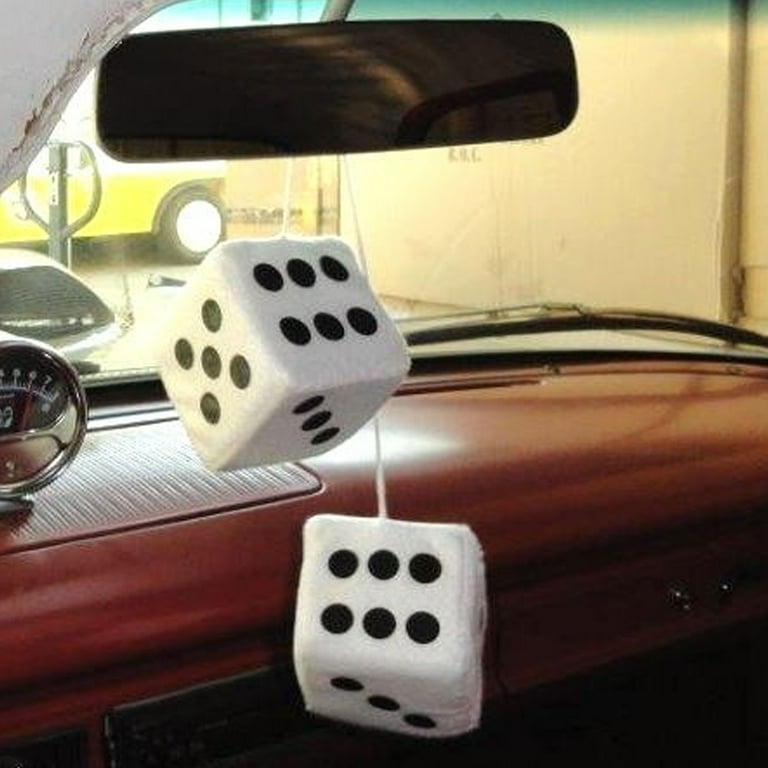The photograph captures the interior of an antique car, focusing on the windshield and the dashboard. The dashboard is colored a rich burgundy or reddish wood, suggesting an older model vehicle. Prominently hanging from the rearview mirror are two plush dice, which are white with black dots; the visible sides show two sixes on the foremost faces, three dots below, and a five on the left side of the upper die. 

Above the dashboard, a gauge with numbers 4 through 8 and a red indicator is noticeable, possibly an RPM meter. Through the windshield, a yellow wall and a yellow vehicle with a white top and black tires are visible, hinting that the car might be parked in a shop. Additional details include a windshield wiper on the right side and what appears to be the handle of a lift jack or machine in the background. The scene is completed with the ground visible outside, which appears to be a light yellow-white color, underscoring that the vehicle is within or adjacent to a structure.